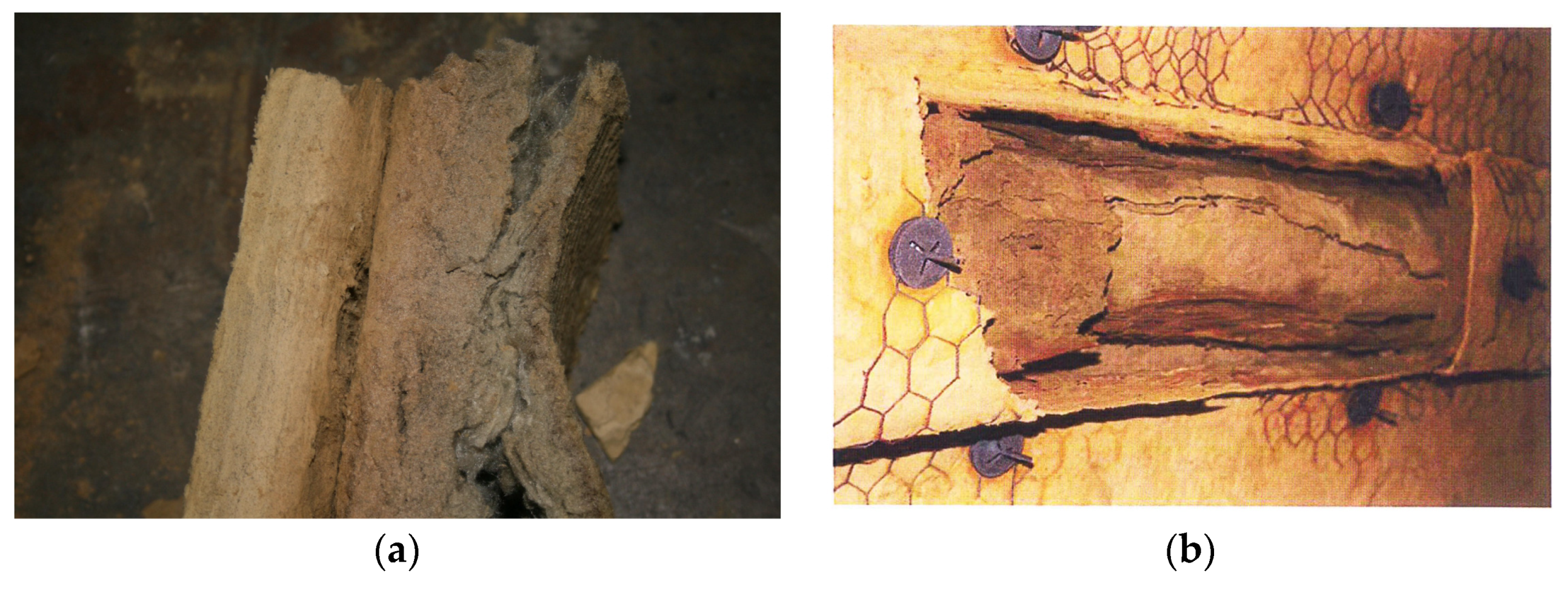The composite image presents three pieces, labeled A and B, that emphasize a theme of decay and exposure. 

In image A, situated on the left, there is a piece of wood with a dark brown background. This piece of wood appears deeply aged, almost disintegrating, with black etchings running down its grain, giving it an abstract, almost painting-like quality. The background transitions into slightly lighter brown tones, creating a subtle contrast that highlights the wood's texture.

Image B, on the right, depicts a brighter, more illuminated scene, suggesting the presence of direct light. Here, a man-made structure appears to be crumbling, revealing what lies beneath its surface. Part of the wall, possibly covered previously by plaster, has eroded away, unveiling a piece of wood at the core. This wooden element is surrounded by a mesh, affixed using various colored fasteners or couplings—purples and blues—strategically placed around the perimeter. The setup also features a counter with layers of chicken wire, further emphasizing the idea of decay and exposure. The detailed environment, marked by these fasteners and the decaying materials, suggests a piece of art that explores themes of deterioration and the revealing of underlying structures.